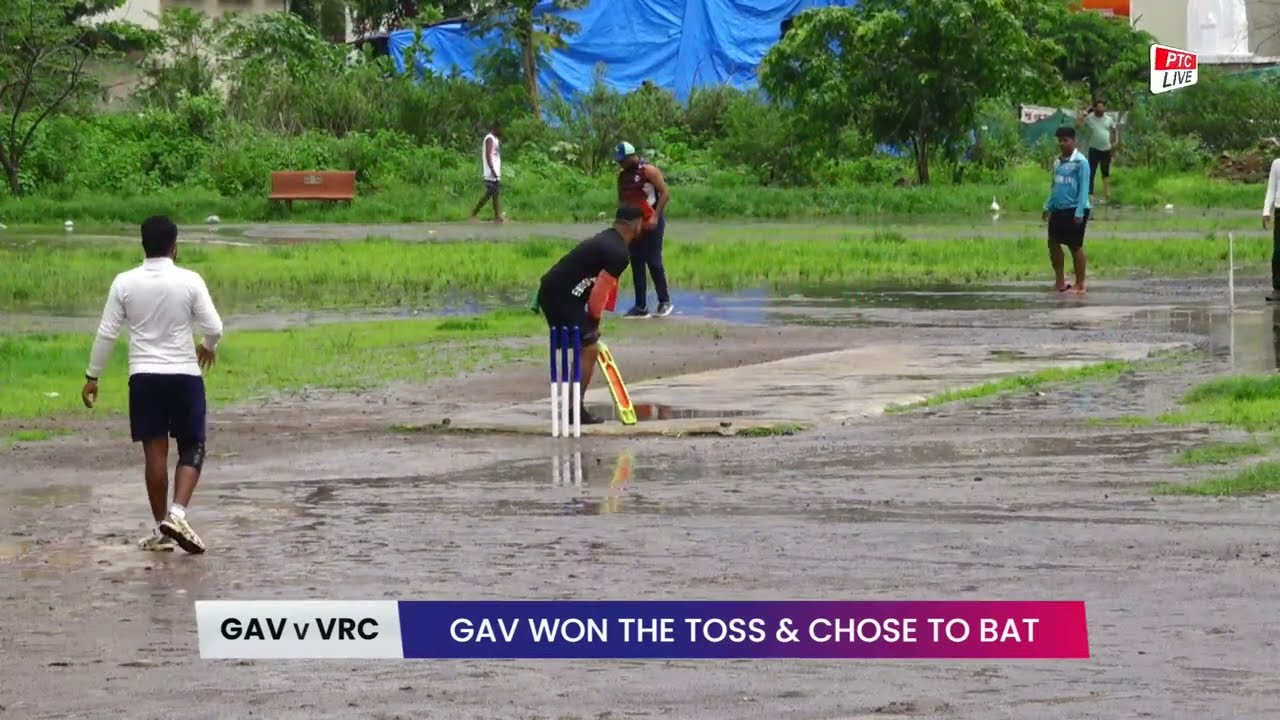The image captures a group of seven individuals playing a game of cricket in a rain-soaked, outdoor setting, likely an overgrown park. The players are dressed in various colorful outfits, including one in navy shorts and a turquoise soccer jersey with a white collar who is poised to pitch. The batter, holding a cricket bat, faces the pitcher intently. The ground is wet, creating numerous puddles, and a light drizzle can be inferred from the setting. Surrounding the players is a grassy field with scattered trees donning green leaves, providing a lush backdrop. The area also contains a blue-tarped building, some ducks wading in a puddle, a brown bench on the right, and a red bench in the upper left corner. Overlaid on the image are captions, including "GAV versus VRC," "GAV won the toss and chose to bat," and "PTC Live," suggesting a live broadcast of the cricket match.